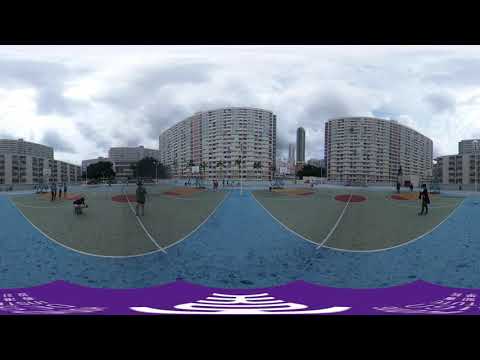The image captures a highly distorted fisheye view of an outdoor recreational area. In the foreground, there is a tennis court and a basketball court, suggesting a multi-purpose sports facility. Several people are visible, engaged in various games. The area is lined with palm trees, hinting at a pool nearby. The scene features a unique blue pathway that curves from the center towards the edges. Highlighted prominently at the bottom is a Photoshop filter effect that mirrors the image, creating a vibrant blue and purple band with unreadable white text.

In the background, a series of buildings stretch across the horizon, resembling apartment complexes or possibly large hotel resorts. These structures include a notable vertical building that stands alone, gray in color. Further behind, additional tall buildings, possibly office structures or skyscrapers, also populate the skyline. The sky is heavily overcast with dark gray clouds, suggesting cold weather. The overall effect contributes to a sense of distortion and surrealism in the photograph.